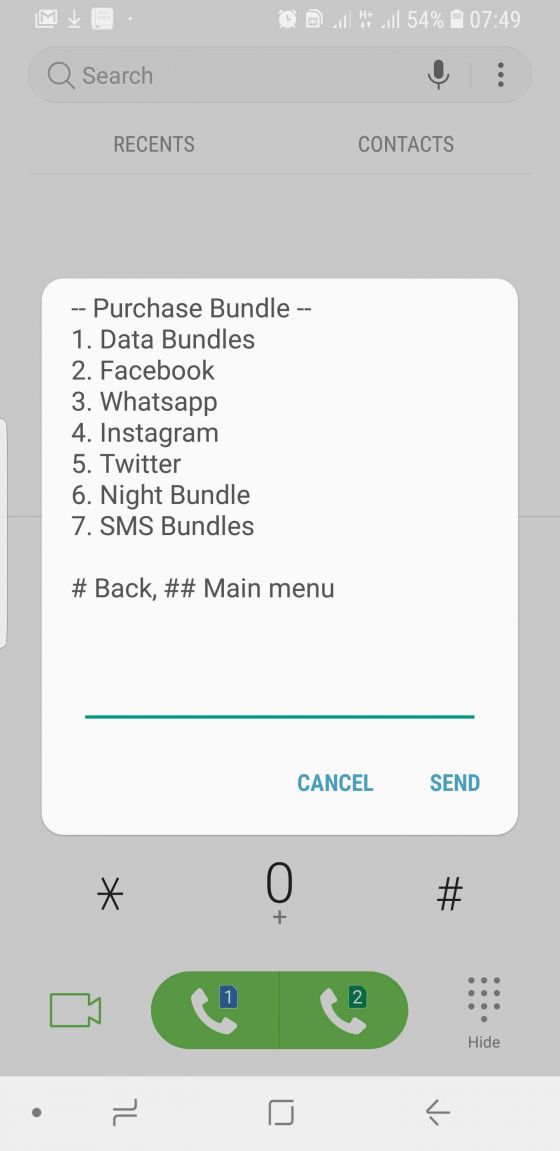This image displays a phone screen featuring a calling app interface. At the top of the screen, icons for the phone, Google Gmail, download, a square symbol, an alarm clock, a SIM card, a network signal with three bars, a full network signal, and a battery indicator showing 54% are visible. The time shown is 7:49. Below these icons is a search bar overlaying a grayed-out background, with a white square prominently displaying "Bundle Purchased." Below this header, there is a list numbered from 1 to 9 with the following entries: 

1. Data Bundles 
2. Facebook 
3. WhatsApp 
4. WhatsApp (again, likely a typographical error in the original list) 
5. Instagram 
6. Twitter 
7. Other Bundles 
8. SMS Bundles
9. Hashtag Bag 

Near the bottom of the screen, a navigation menu displays two options: "Cancel" and "Send," both highlighted in blue.